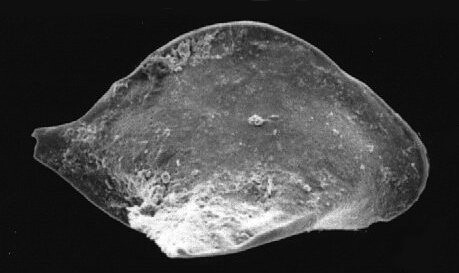This image, captured under a microscope, features a central, irregularly shaped object set against an entirely black background. The object, which resembles a rough-surfaced microorganism or a rock, occupies most of the frame's width of approximately 3 inches and length of around 4 inches. It has an asymmetrical, somewhat oblong shape, wider at the top and tapering on the left and right sides, most notably on the right. The bottom edge extends into a fin-like point. The object displays varying textures, with particularly rough areas near the bottom fin. Intriguingly, there's a round, rough patch in the center resembling an eye, though it's unlikely to be one if this is indeed a microorganism or rock. The grayscale tones accentuate the rough textures and wavy patterns, especially at the lower part where a lighter shading contrasts with the darker hues of the object. The stark black background further isolates the object, emphasizing its detailed and rough structure.